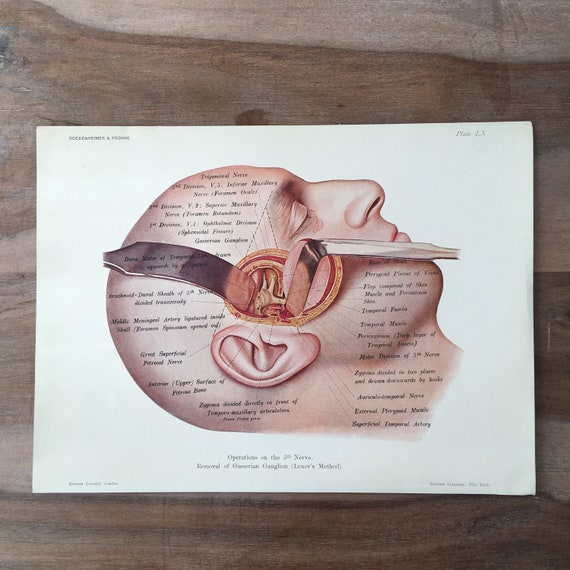This image captures an intricately detailed medical diagram laid flat on an aged wooden table, displaying a faded grain texture. The diagram itself is drawn on a white piece of paper, rendered in a horizontal rectangular format. It depicts a bald male figure with closed eyes, suggesting he is lying down and possibly asleep. The top of the man's skull is shown with an opening that reveals the inner structures of the head. This opening is located prominently between the ear and the end of the eye socket, exposing a network of nerves and inner facial components in varying shades of pink and red.

Several sharp instruments are illustrated pulling back the skin to provide a clear view of these inner workings. Multiple annotations are present, indicated by black lines and dots pointing to different parts of the exposed area, explaining the various components. Text accompanying the drawing includes a note reading "operation of the fifth nerve." The entirety of the diagram and its details combine to provide an insightful look into the complex anatomy beneath the face, set against a visually contrasting background composed of varying shades of brown on the wooden table.